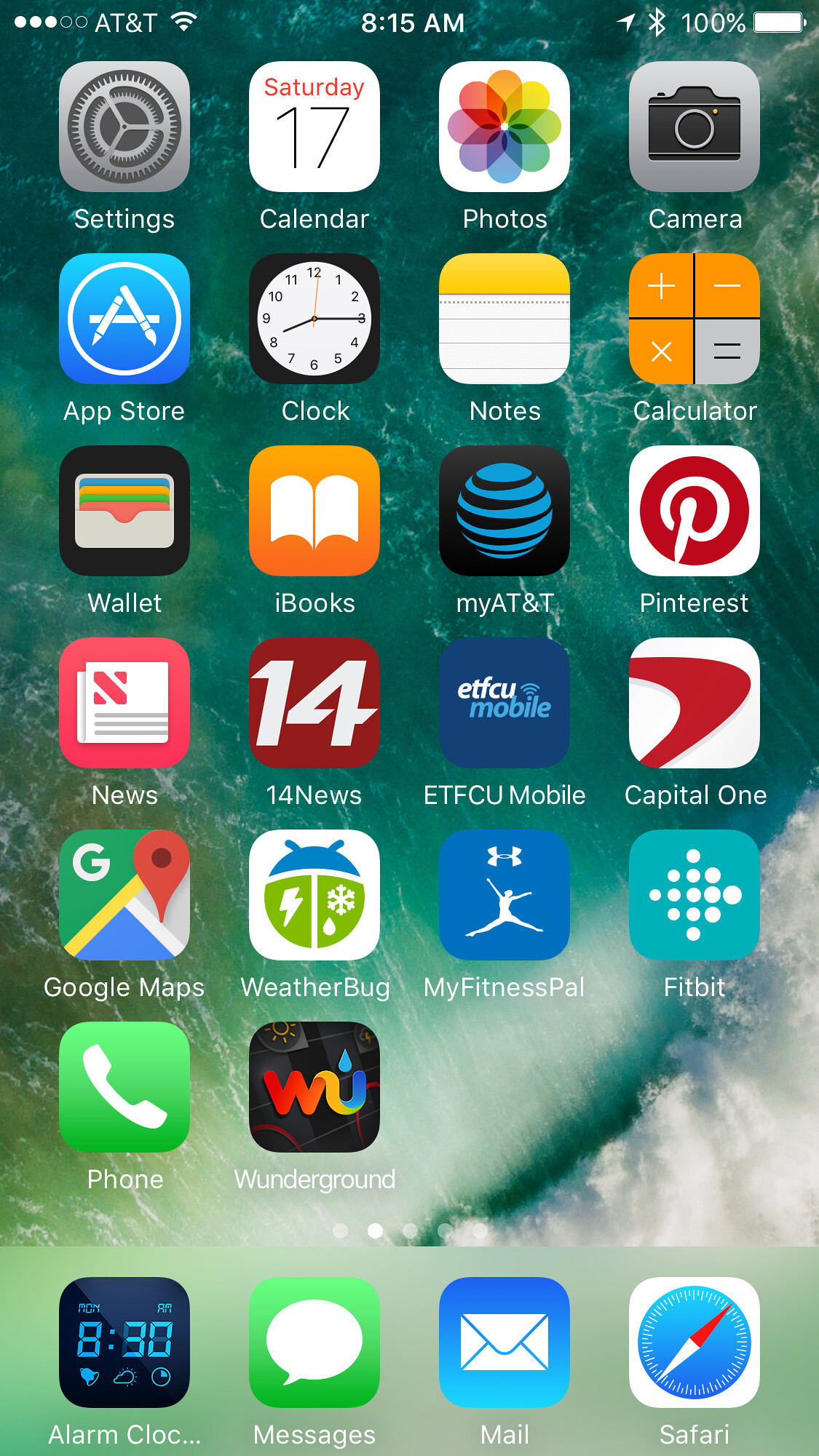**Detailed Description of a Smartphone's Home Screen:**

The screenshot captures the home page of a smartphone, set against a serene underwater background. The wallpaper displays a deep, greenish-blue ocean that gradients down to about two-thirds of the left side of the screen, and then arches slightly upward to the right, culminating in frothy white waves at the bottom.

In the status bar located at the top of the screen:
- The upper left corner features five dots, with three lit white, indicating moderate signal strength, followed by "AT&T" in white text.
- Further to the right, there's a Wi-Fi icon showing full connection.
- Centered at the top, the time reads "8:15 AM."
- On the upper right side, there is an arrow pointing up and to the right (likely an upload indicator), followed by the Bluetooth icon.
- Adjacent to this is the battery percentage displayed at "100%", and next to it on the far right is the battery icon itself.

Arranged in a grid format are several apps:
- **First Row (left to right):** Settings, Calendar, Photos, Camera.
- **Second Row (left to right):** App Store, Clock, Notes, Calculator.
- **Third Row (left to right):** Wallet, iBooks, MyAT&T.
- **Fourth Row (left to right):** News, 14 News, ETFCUMobile, Capital One.
- **Fifth Row (left to right):** Google Maps, WeatherBug, MyFitnessPal, Fitbit.
- **Sixth Row (left to right):** Phone, Wunderground (WunderGround weather app).

At the bottom dock:
- **Left to right:** Alarm Clock, Messages, Email, Safari browser.

The organization of the apps on the home screen, combined with the tranquil oceanic wallpaper, suggests a user who values both functionality and aesthetic serenity.